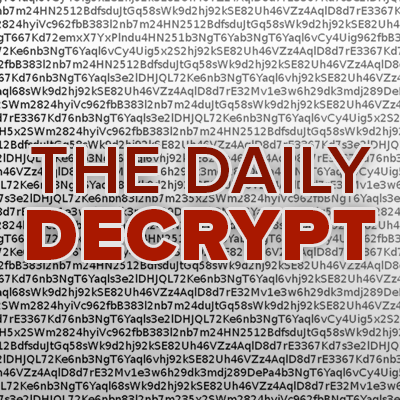The image features a square format with an intricate background composed of indiscernible rows of letters and numbers in black font, creating a pattern of seemingly random gibberish on a white backdrop. This text engulfs the entire image, extending from edge to edge without any discernible order. Centrally placed on this chaotic background are two lines of bold red text with a white outline. The top line reads "THE DAILY" in slightly darker red capital letters, while beneath it, in a slightly lighter shade of red, the text spells out "D-E-C-R-Y-P-T" in larger capital letters.